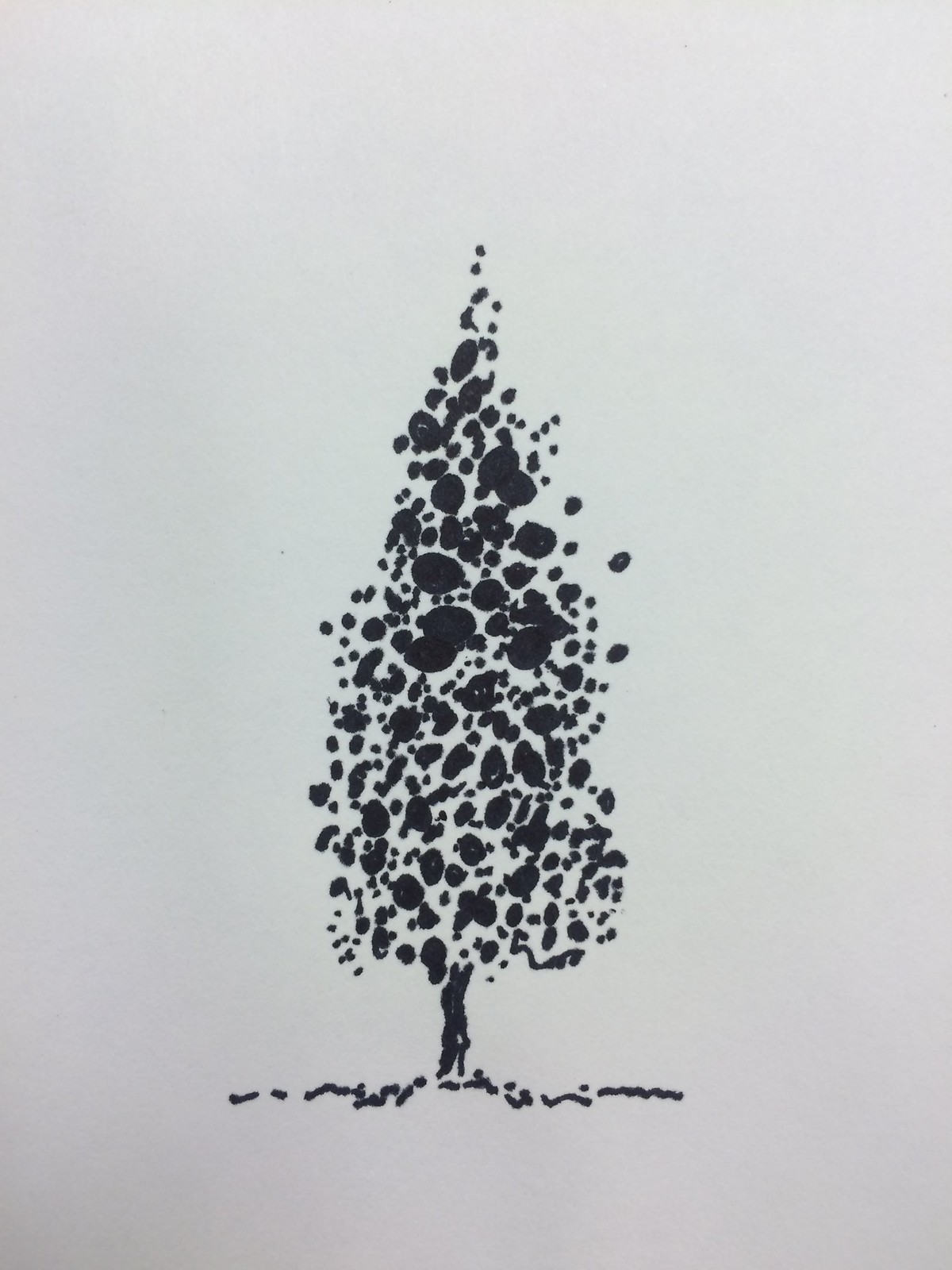This artwork features a tree composed predominantly of different-sized ink dots and a few lines, all in black. The tree’s shape resembles a Christmas tree, broad at the base and tapering to a point at the top. It is set against a gray background that exhibits an ombre effect, transitioning from a darker gray at the bottom to a lighter gray at the top. The ground is represented by a series of ink blots and squiggles at the base, with a line suggesting the tree trunk. The entire composition, created with black ink on gray paper, conveys a blend of painting and drawing through its abstract, minimalist dot-and-line structure.